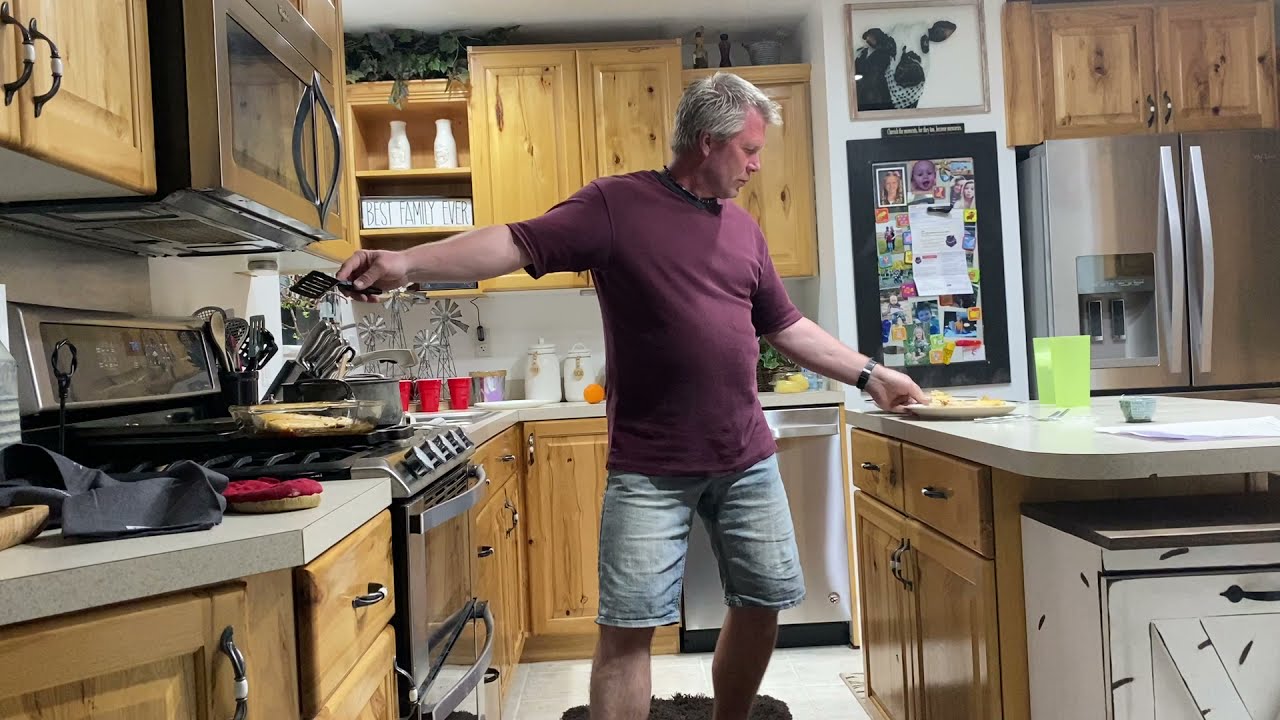**Photograph Description:**

This detailed photograph captures a middle-aged man, likely in his late 40s or 50s, standing in the middle of an old-fashioned kitchen. He's wearing a purple t-shirt and light blue denim shorts, known as jorts. His hair is blondish with noticeable graying, and he has a pale complexion. The man is multitasking—his left hand holds a plate overflowing with food, which he's placing on a wooden table to his right. Meanwhile, his right hand wields a spatula over a cooktop, suggesting he is preparing a meal.

Surrounding him is a cozy, well-used kitchen with numerous wooden cabinets, which store a variety of utensils. There's an aluminum steel refrigerator adorned with colorful post-it notes and a pinboard with family photos, including images of babies and a charming picture of a cow. The countertops, which appear to be made of Formica, are accented by two yellow glasses. Under his feet, a black fuzzy rug adds a homely touch to the scene. A glass casserole dish from which he's taking food, labeled "Best Family Ever" in Sharpie, signifies the familial warmth of this household.